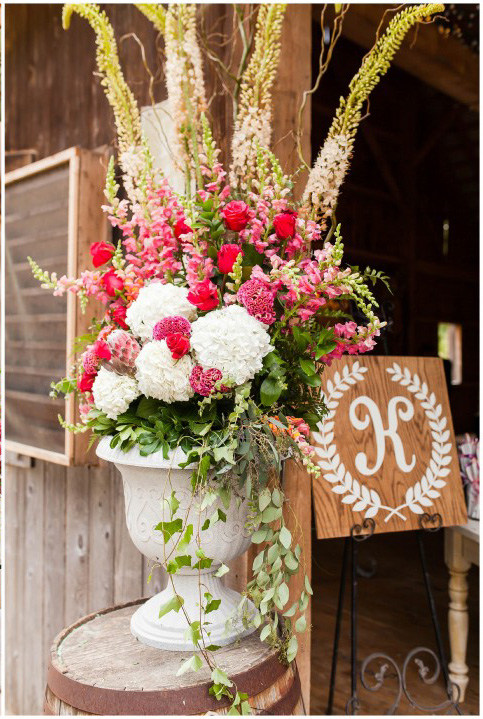The image captures the entrance of a weather-beaten wooden building, characterized by visible grooves, cracks, and nail marks in the wooden planks and floors. The interior is dimly lit, accentuated by light streaming in from outside. Dominating the scene is a decorative floral arrangement positioned atop a wooden barrel near the open doorway. The large, white ceramic planter, shaped like a wine goblet, holds an elaborate mix of flowers: pure white hydrangeas, pink and red roses, fuchsia blooms, and vivid yellow flowers with green stalks. Cascading ivy and green tendrils add to the lushness of the display. Close to this arrangement is a square wooden sign resting on a stand, featuring an ornamental "K" encircled by a near-complete wreath of white leaves.